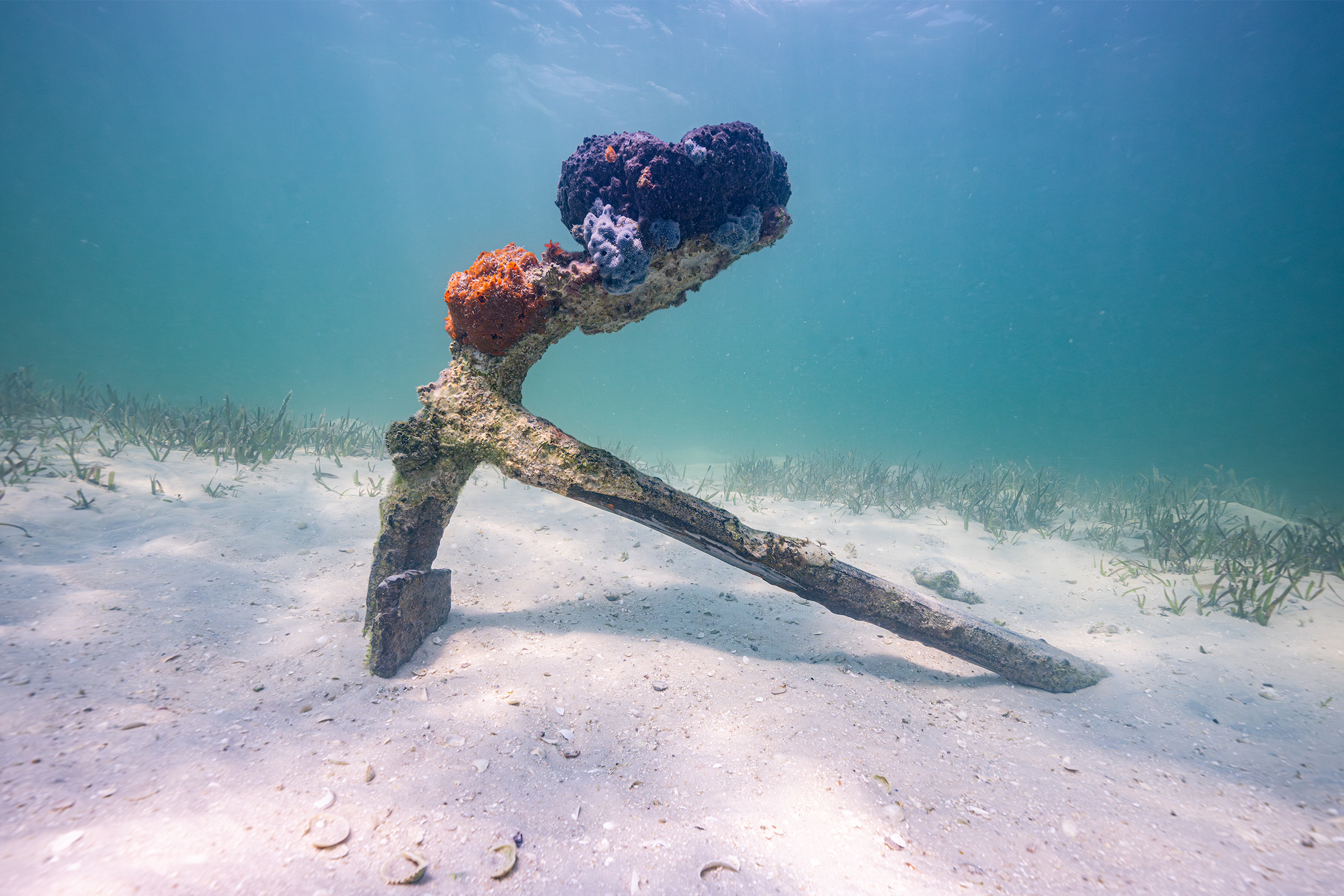This captivating underwater photograph showcases a rusted, old ship’s anchor partially buried on a bright, sandy seafloor scattered with shells and tufts of green seagrass. The anchor, prominently placed front and center, is heavily corroded and encrusted with vibrant corals and barnacles, displaying hues of red, orange, purple, and blue. The water surrounding the scene is a clear, medium to deep blue, with sunlight streaming down and creating an almost magical atmosphere, indicating shallow, warm tropical waters. The surface of the ocean is visible in the background, with subtle ripples adding to the serene yet mysterious ambiance of the image.